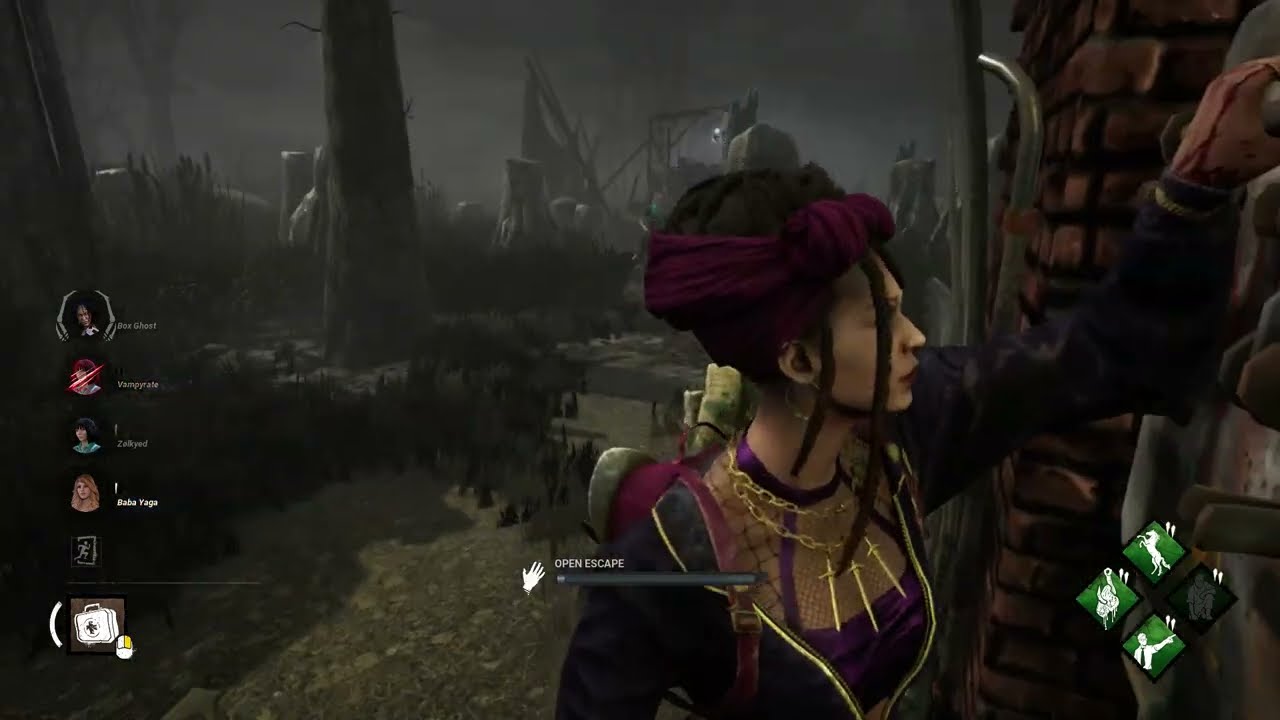The image appears to be a detailed screenshot from a video game featuring the main character, a woman of white complexion with her hair styled in dreadlocks pulled up into a top bun, adorned with a few loose strands and a burgundy scarf tied into a bow at the front. She also wears a hoop earring and a distinctive purple dress featuring mesh fabric near the chest. Over the dress, she sports a jacket, and a pink and gray backpack is visible on her back. A gold chain necklace with three sword pendants dangles around her neck. Her right hand, which has some visible blood on it, reaches towards a door or similar object. The scene is set outdoors in a predominantly gray, forested area with cut-down trees and some bushes and rocks, creating an apocalyptic atmosphere highlighted by dark, rubble-filled surroundings. Various gameplay symbols and controls are displayed on the screen, including icons on the left and right, and a health bar in the middle with the text "open escape." The entire scene conveys a sense of destruction and survival.